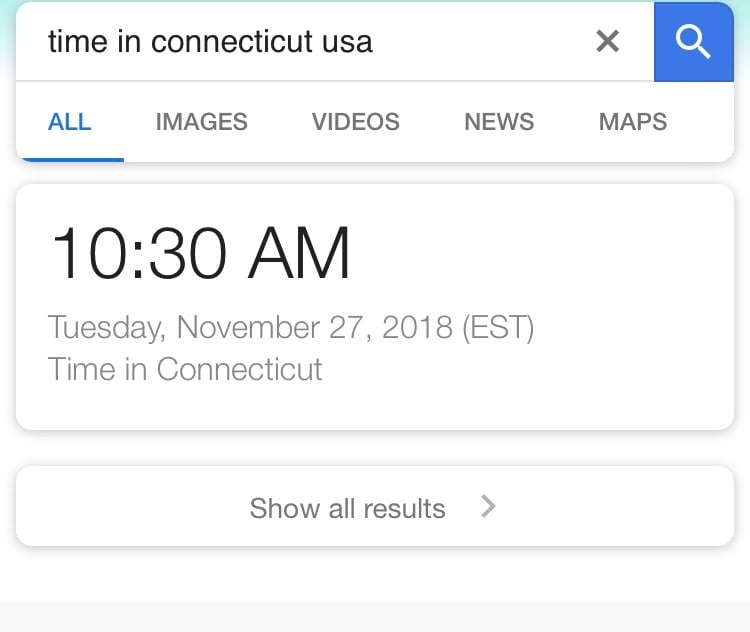This screenshot features a snippet from a search engine, likely Google, depicting information about the current time in Connecticut, USA. At the top of the image is a search bar with the query "time in Connecticut, USA" entered. Adjacent to the search bar on the right, there is a grey "X" icon followed by a blue square with a white magnifying glass icon, commonly used to execute the search. 

Directly beneath the search bar, a navigation menu presents five options: All, Images, Videos, News, and Maps. The "All" option is highlighted in blue text with a blue underline, indicating the current selection.

Further down the screen, a prominent white rectangular box displays the current time as "10:30 AM" in large black text. Below this, the date "Tuesday, November 27, 2018" is provided, followed by “(EST)” which denotes the Eastern Standard Time zone. An additional line of text reiterates "Time in Connecticut," and a prompt at the bottom of this section reads "Show all results."